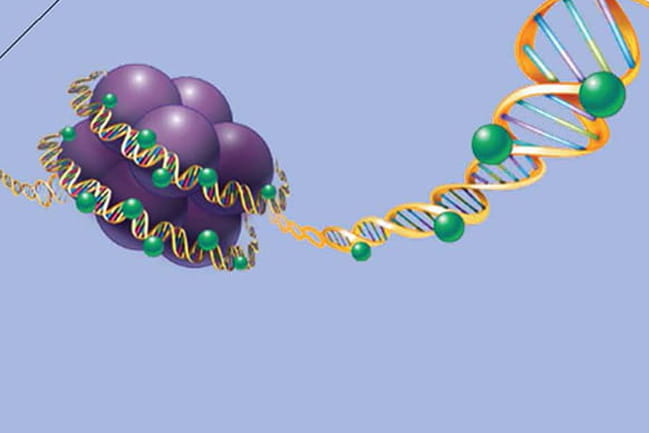This detailed diagram illustration of a biological material showcases an intricate interaction between DNA and cellular structures. On the left, a cluster of eight large dark purple spheres, resembling balloons, is prominently featured. These spheres are enveloped by a double helix structure, depicted in gold, which wraps around the purple cluster at two distinct points before extending out to the right. The DNA itself is highlighted by gold outer strands that crisscross and intertwine, with lines between them appearing in various colors: pink, blue, green, yellow, white, and purple, which repeat in a consistent pattern.

In addition to the large purple spheres, smaller green spheres are seen rotating from left to right at each crossover of the gold DNA strands, adding a dynamic element to the illustration. The background is primarily light periwinkle or light blue in color, creating a cool, serene backdrop for the complex biological material. Additionally, in the top left corner, a black strip runs across, further framing the central diagram.